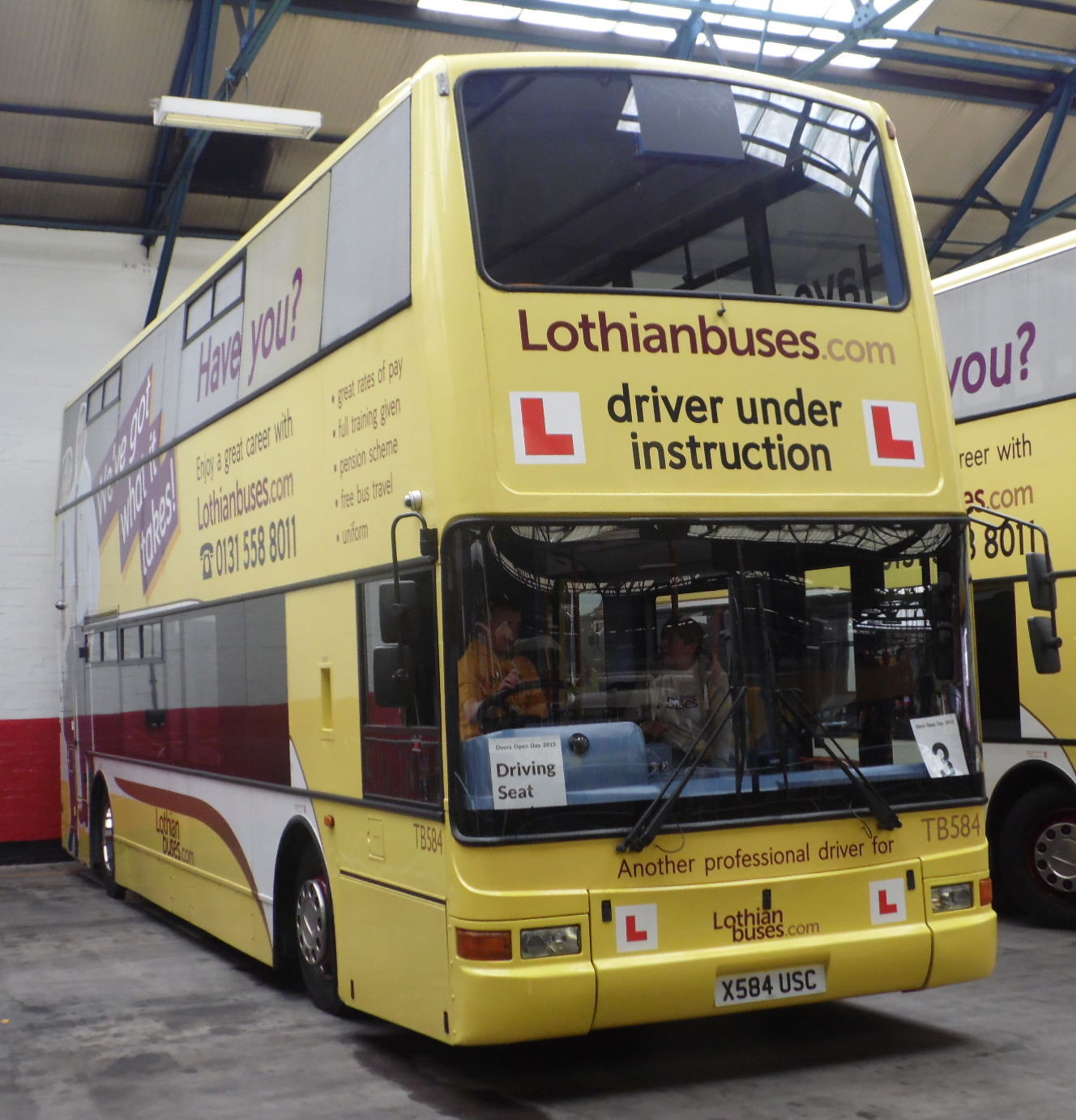The image depicts two parked double-decker buses inside a large garage or under an awning, in front of a white wall with a red stripe. The buses are primarily canary yellow with dark tinted windows. The bus in the foreground prominently displays "LothianBuses.com" in maroon text below the front second-floor window and above the driver on the right-hand side. The front bus also features black text below the windshield, reading "Another Professional Driver 4 TB-584," and further down, "LothianBuses.com" between the headlights. Notably, "Driver Under Instruction" is written in black text with a red "L" in a white box on either side. Side advertising includes slogans like "Have you got what it takes?" and "Enjoy a great career with LothianBuses.com," alongside bullet points listing benefits such as great pay, full training, pension schemes, and free bus travel. The driver in the foreground bus wears a yellow long-sleeve shirt. A sliver of the second bus to the right is visible, marked similarly but mostly obscured.